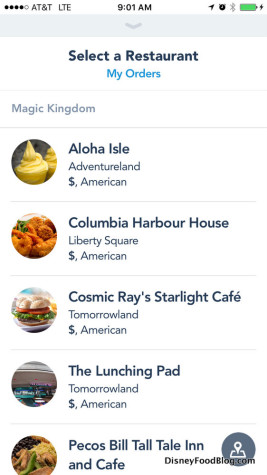This is a detailed screenshot taken from a cell phone. The device is connected to AT&T network, showing LTE service at 9:01 a.m. The status bar at the top displays several icons including a fully charged battery symbol, which is colored green. Below the status bar, the screen shows a heading "Select a Restaurant," followed by a blue-colored link that reads "My Orders," allowing users to view their order history. In the upper left corner, "Magic Kingdom" is displayed in a smaller, grayish font.

Five profile icons associated with different dining options are listed vertically on the screen. These are accompanied by corresponding images and names:

1. An ice cream cone icon within a circle labeled "Aloha Isle Adventureland," described as an "American S."
2. A food picture labeled "Columbia Harbor House."
3. An image labeled "Cosmic Ray Starlight Cafe."
4. Another icon for "The Launching Pad."
5. A final image labeled "Pecos Bill Tall Tale Inn and Cafe."

This descriptive caption provides a detailed overview of what is visible on the phone's display screen.